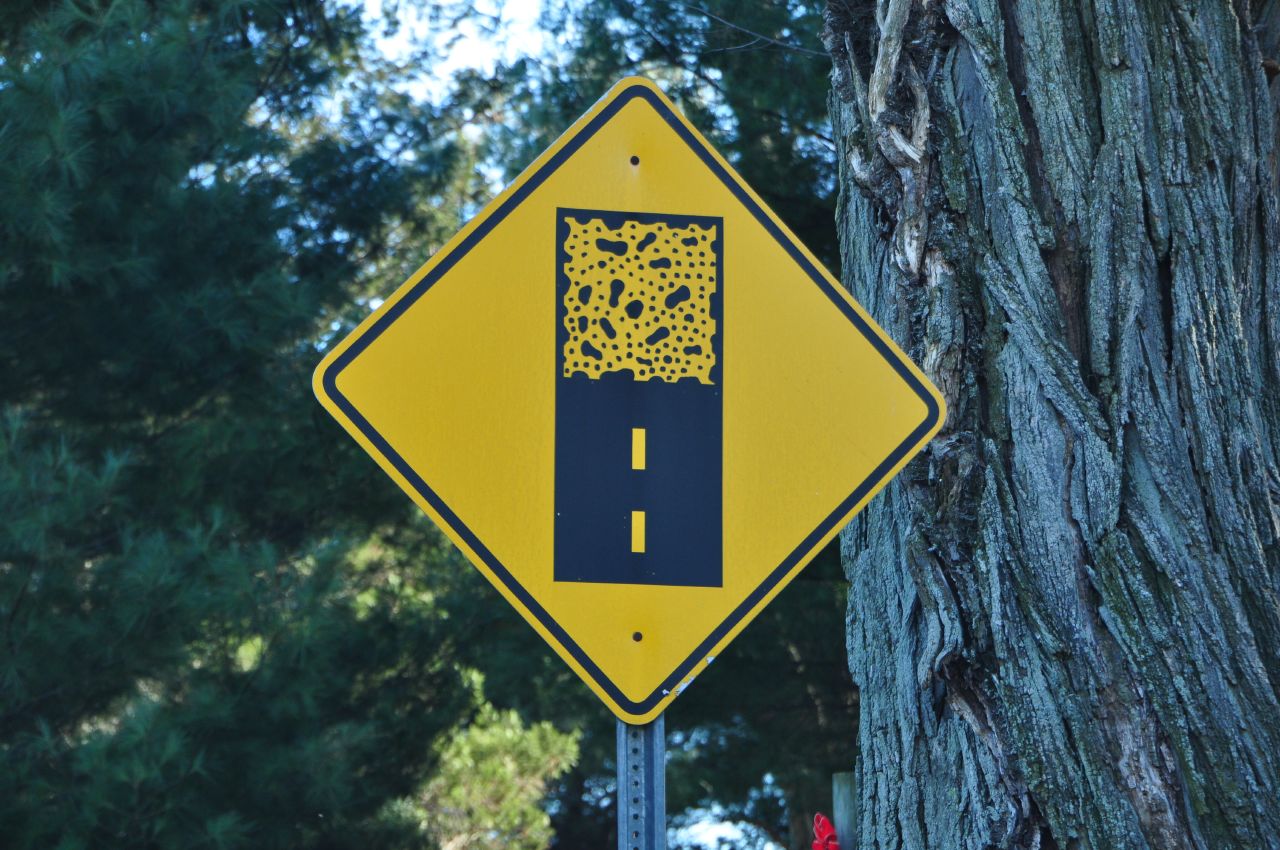This photo captures a unique yellow diamond-shaped roadside sign taken during the daytime. The sign is unusual and features an illustration of an ascending road with what appears to be footprints or some form of irregular markings on the top half. The sign's purpose is unclear. Positioned to the right of the sign is a large tree, with a portion of its bark visible in the frame. In the background to the left, a dense cluster of green pine trees completes the natural setting.